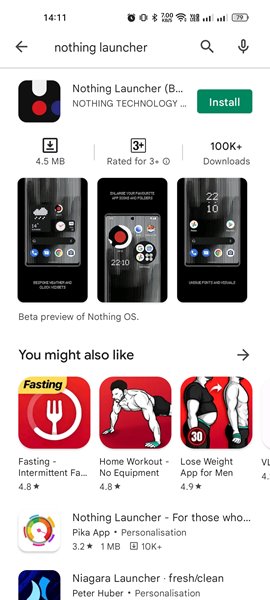The image displays various on-screen elements typically found on a smartphone interface. The top bar features the time "14:11," along with icons for a clock, vibrating mode, a Bluetooth symbol, WiFi connection, another signal indicator, and a 79% battery level. Below, there is a left arrow, a search bar with a magnifying glass icon, a microphone, and various other icons. 

The centerpiece shows a layered arrangement of interfaces: 
- A black icon towards the center.
- A white text overlay near the top.
- A blue half-circle on the right.
- Numerous references to "Nothing Launcher" and "Nothing Technology."
- Green "Install" button with details like “4.5 MB” and “3+” indicating the app's size and content rating respectively. 
- The mention "100K+ downloads."

On the left side, a smartphone is depicted with a square background displaying various elements. This includes more blue tones, a Google search bar, a camera icon, and a text section.

Further down, another smartphone illustration indicates a "Beta Preview" for some applications. Specific suggestions such as:
- A green app icon labeled "You Might Also Like."
- A red square icon, yellow at the top left.

There is also an app for fasting with a focus on intermittent fasting rated 4.8 stars, depicted by a muscular person doing push-ups, indicating a home workout without equipment. Another app is portrayed with a 4.8-star rating, showing a transition from a glutton to a muscly figure, suggesting weight loss benefits.

Additional app icons include:
- The "Nothing Launcher" emphasizing customization for users.
- An app labeled "Pika App" with a personalization rating of 3.2 stars and a size of 1 MB with over 10,000 downloads. 

The bottom left shows a blue square, referring to "Niagara Launcher – Fresh, Beta, Hyper-personalization."

Overall, the image conveys a complex smartphone interface with numerous apps, functionalities, and personalized customization options, highlighting their features and user ratings.